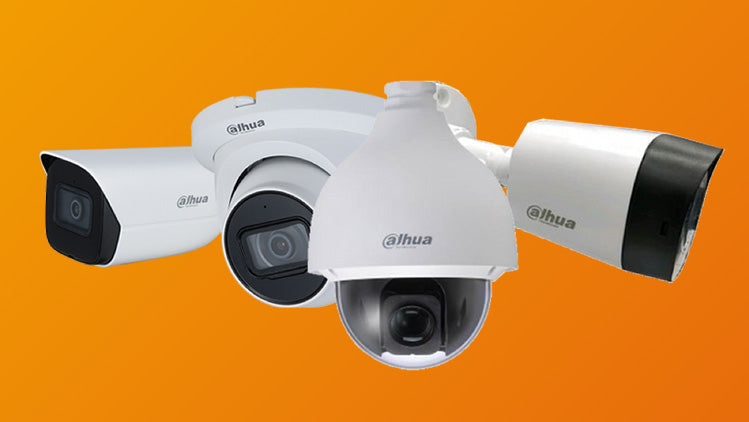The image displays a sophisticated security camera setup against an abstract orange background with a gradient effect, transitioning from a lighter orange in the upper left corner to a darker orange in the bottom right. Central to the image is a white security device that appears to be mountable, possibly on a ceiling or wall, featuring a circular base that suggests an open top. The unit comprises two lights and two recessed cameras, each with a black covering and clear lens. A light sensor is present to activate the lights when motion is detected. The brand "Alhua" is prominently displayed in gray text with a swirling curve around the 'A' on each component. The cameras and lights extend outward: one light and one camera to the left, one light and one camera to the right, and two more cameras projecting frontward and slightly to the front left, completing this detailed and functional security system.